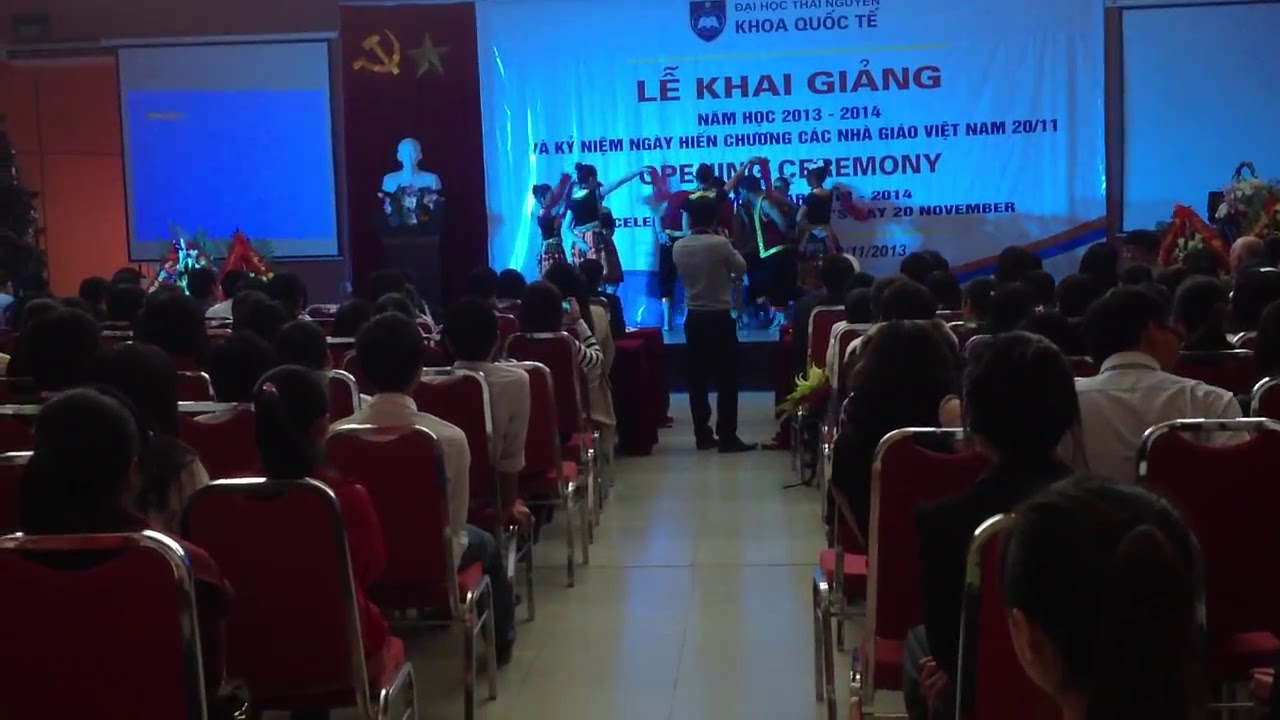The image captures a horizontally aligned rectangular setting during an opening ceremony in Vietnam, dated November 20, 2014. The auditorium is filled with formally dressed attendees sitting in red chairs with silver borders and legs, extending down an aisle from which we view the backs of their heads. Most chairs are occupied, indicating a full house. Men in the audience are seen wearing white long-sleeve dress shirts with collars.

At the far end of the aisle, a modestly sized stage is adorned with various elements. Dominating the backdrop is a large banner bearing the words “Le Kai Jiang,” and the phrase “Opening Ceremony” in English among other Vietnamese inscriptions. The walls are painted red and feature prominent symbols, including a star and the hammer-and-sickle emblem of the Soviet Union, alongside a white bust near the stage—a likely nod to Vietnamese heritage or historical figures.

A man stands in the aisle, positioned in front of the attendees but not on the stage, dressed in black slacks and a long-sleeve dress shirt. Additionally, he appears to be photographing the event, suggesting he is capturing moments of what seems to be a dance performance by students in costume on the stage. The scene, enriched with intricate cultural and ceremonial elements, indicates a significant and formal event in Vietnam.